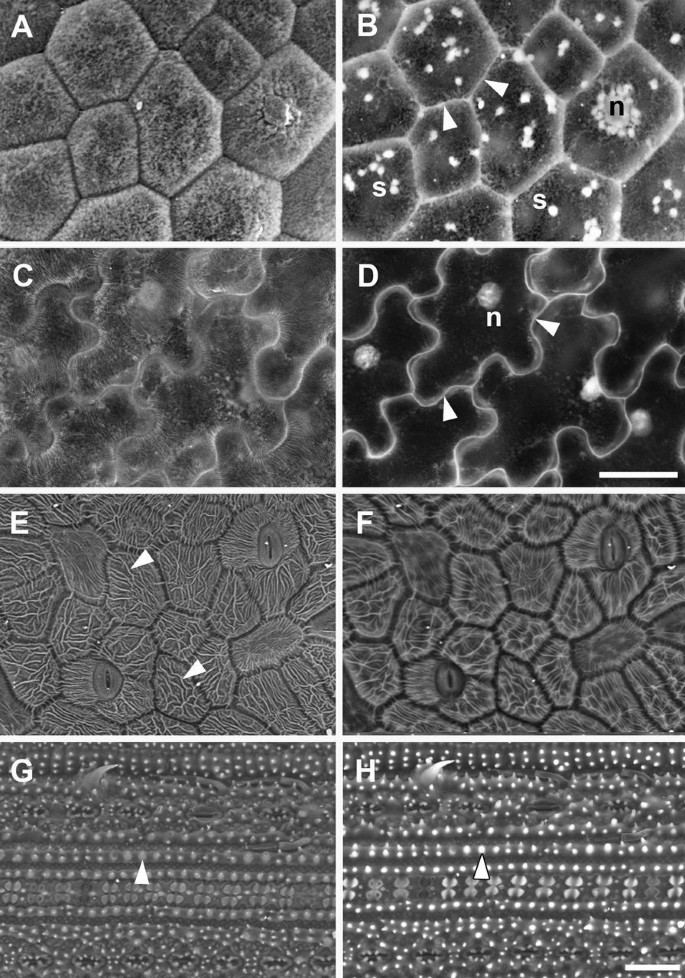This image displays a detailed array of eight microscopic close-ups, labeled A to H, meticulously organized in two columns of four. Each slide presents unique structural formations observed using an electronic microscope, all rendered in varying shades of gray, black, and white tones. 

Slide A shows a honeycomb-like pattern with dimples in the centers. Slide B features a similar honeycomb structure, only in dark gray with black splotches, white dots, and two central triangles. To the right of these in particular formations, there are clusters of white dots, labeled N and S respectively.

Slide C, located on the second row, exhibits squiggly lines resembling slashed raindrops on glass. Next to it, slide D illustrates darker puzzle-like pieces, annotated with arrows pointing to N and D in the upper left corner. Two dark gray circles are positioned within the slide – one between the D and the triangle, and another by the N.

Moving to the row labeled E, this slide features eye-like shapes in the lower left and upper right corners, with thin black circles as pupils amidst various triangles. Slide F to its right zooms in on this honeycomb structure, showing similar eye-like designs with an F marked in the top left corner.

The final row contains slide G, displaying wavy dots resembling beads flowing in multiple rivers, some orderly and others dispersed. Slide H, adjacent to G, presents a more defined formation, with all beads illuminated, forming a river-like rectangle with lily pad-like structures.

Overall, the intricate annotations and differing degrees of magnification highlight specific points of interest in these scientific samples, providing an intriguing glimpse into their microscopic complexity.